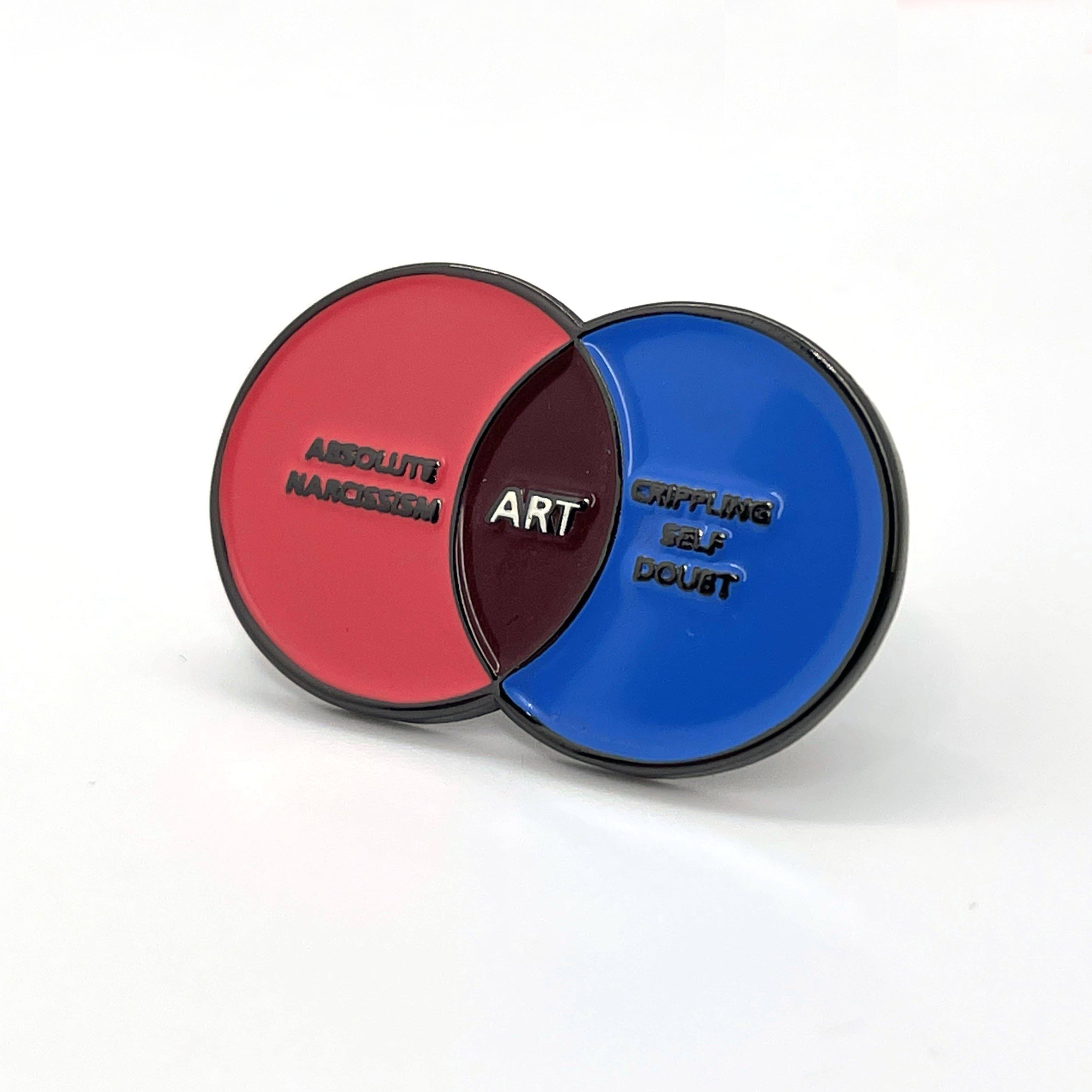This photograph captures a detailed sculpture of a Venn diagram, crafted from a material that gives it a glassy, ceramic-like appearance. The sculpture consists of two overlapping circles, each outlined in black. The left circle is a vivid red with the black text "Absolute Narcissism," while the right circle is a striking blue with the black text "Crippling Self-Doubt." Where these two circles intersect, they form a purple, football-shaped area that features the word "Art" in white text. The entire piece is set against a plain white background, emphasizing its three-dimensional quality and its nature as a unique art piece.